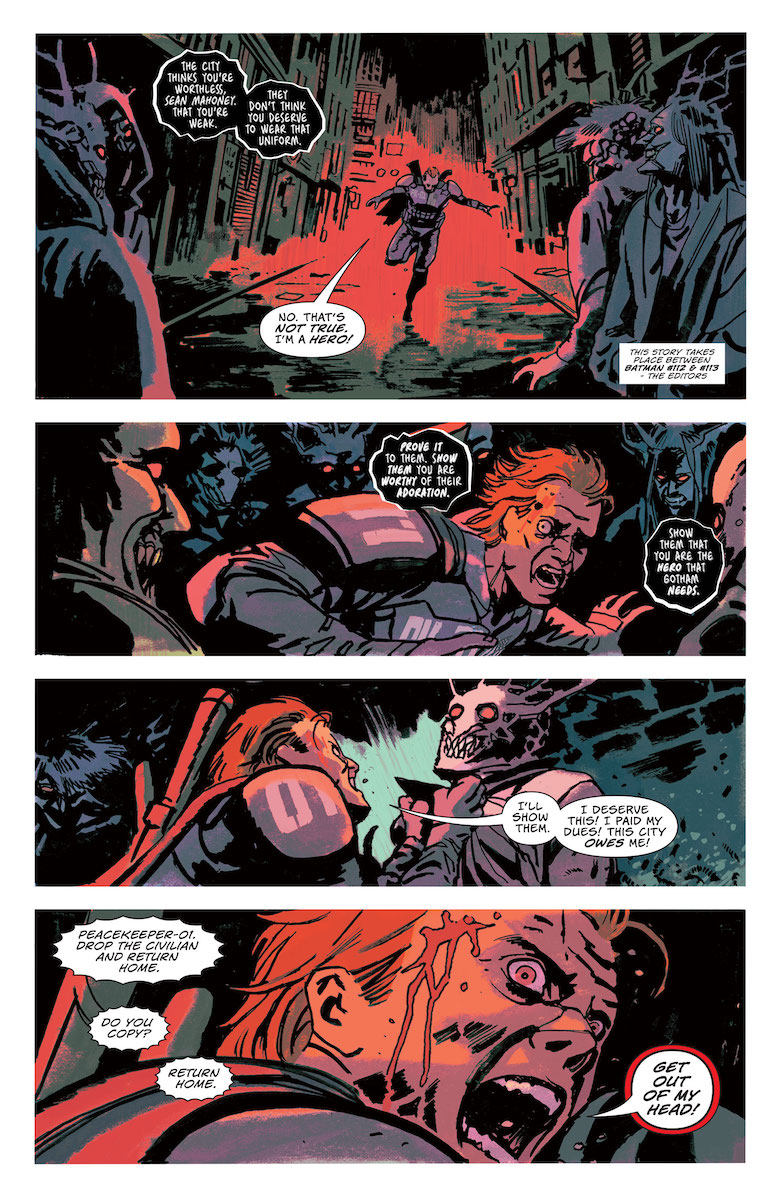The image features four consecutive panels from a graphic novel that takes place in the dark, brooding cityscape of Gotham, predominantly illustrated in deep hues of dark green, gray, red, and black. The narrative is tightly interwoven with intense action and psychological tension. It features Sean Mahoney, also known as Peacekeeper-01, who appears mentally tormented and grappling with a sinister inner voice. The scenes unfold with Mahoney depicted in various states of psychological distress, starting with him running amid eerie, shadowy figures, which voice the city's disdain: "The city thinks you're worthless, Sean Mahoney, that you're weak. They don't think you deserve to wear that uniform." Mahoney fights back, determined, "No, that's not true! I'm a hero!" In subsequent panels, he becomes increasingly desperate, exclaiming, "I'll show them. I deserve this. I paid my dues. This city owes me." His confrontation reaches a climax as he aggressively grabs a skull-faced figure, all while the command "Peacekeeper-01, drop the civilian and return home. Do you copy? Return home," is broadcast. Mahoney, in a panic-stricken, agitated state with wide, frantic eyes, screams, "Get out of my head!" The story is placed between Batman issues 112 and 113, adding contextual depth to the unfolding drama.